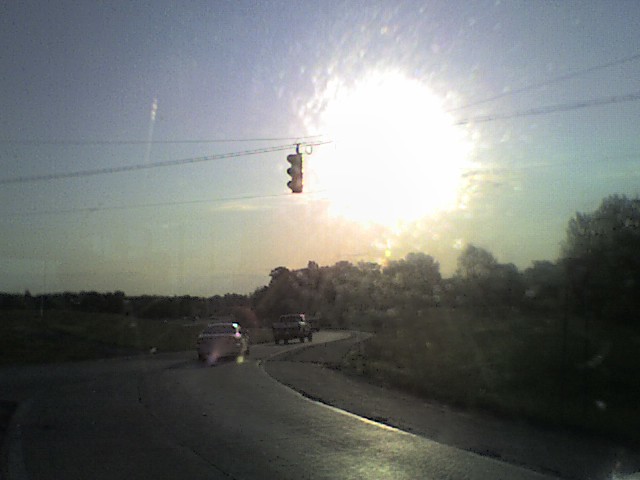A winding road curves gently to the right, with two cars traveling along it—one black and one silver. A noticeable plume of smoke trails from the exhaust of the silver car, drifting across the scene. Overhead, traffic lights suggest the presence of a nearby junction. The sides of the road are lined with lush grassy verges and hedgerows, framed by a backdrop of tall trees. The sky above is a vibrant blue, partially obscured by a cloud that has the sun hidden behind it, casting a soft white glow with a hint of pink beneath.